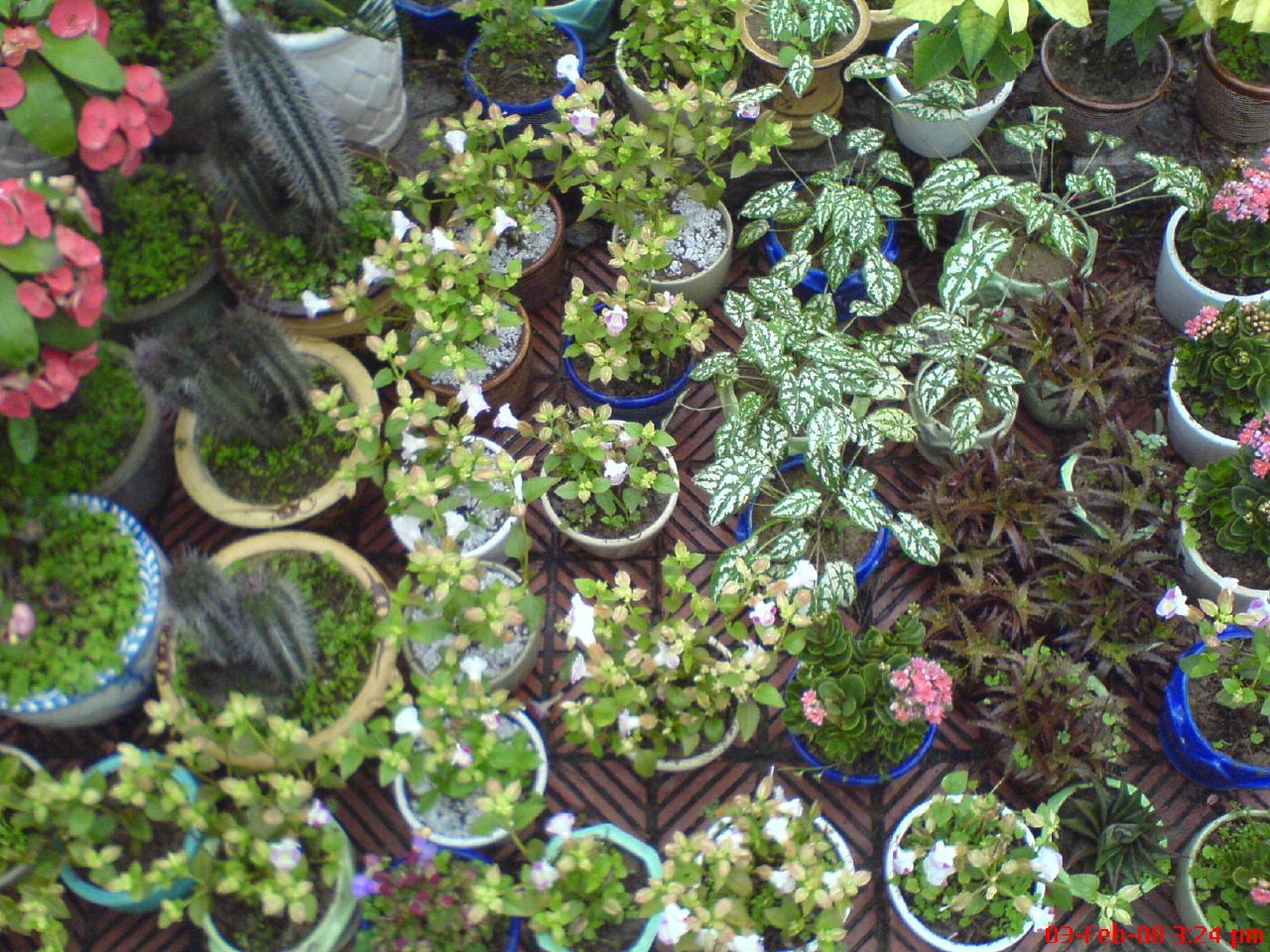The image depicts a wooden terrace densely covered with an assortment of potted plants arranged in a grid-like pattern on a black and brown striped tile surface. In the upper left corner, several pots feature large green leaves with pink blossoms, possibly geraniums. Adjacent to these are three yellow pots housing tall cacti with spiny exteriors. The lower left corner showcases three pots filled with greenery. Across the bottom, starting from the right corner and curving around, are rows of pots containing white petunias in variously colored containers.

Central to the image, some pots display dark green and white variegated leaves, possibly of the Wandering Jew variety. Additionally, there are groups of pots with pink geraniums, notably three white pots on the far right. Scattered between these are several pots with dark-colored leaves and other plants showing bits of white. Despite the diversity in plant types and colors, most pots are blue or white, adding to the coherence of the arrangement. A date, partially visible as "7.24 PM," marks the time when this vibrant garden scene was captured.